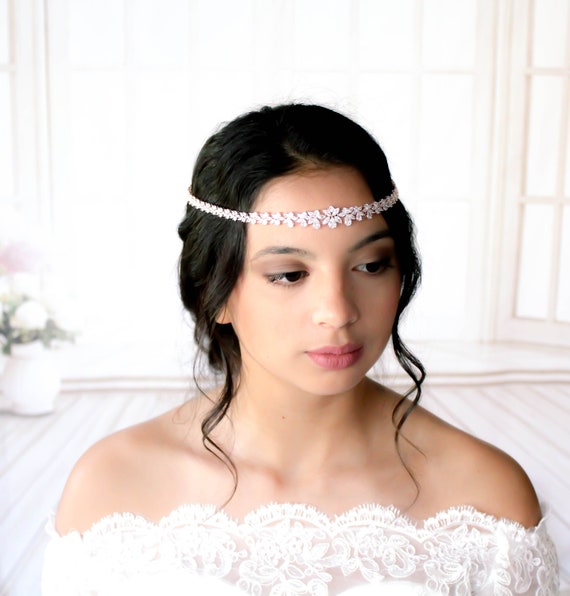The image showcases a bride in a bright, all-white room bathed in natural light. She wears a strapless, off-the-shoulder white gown with a scalloped lace trim, complemented by a floral and jeweled headband that wraps around her forehead. Her long, dark hair is pulled back, with two tendrils slightly curled, falling just below her ears. The bride's eyes are dark, and her complexion is tan, enhanced with minimal makeup featuring light brown eyeshadow and rose-petal pink lipstick. She is gazing downwards and to the right, with an expression that appears somewhat indifferent or contemplative. The room has white wood plank flooring and bright windows, creating a soft, luminous backdrop. In the background, there are white flowers in a vase that reveal green stems, adding subtle color to the scene. Additionally, there is a touch of pink in one of the flower bunches, emphasizing the bridal theme.